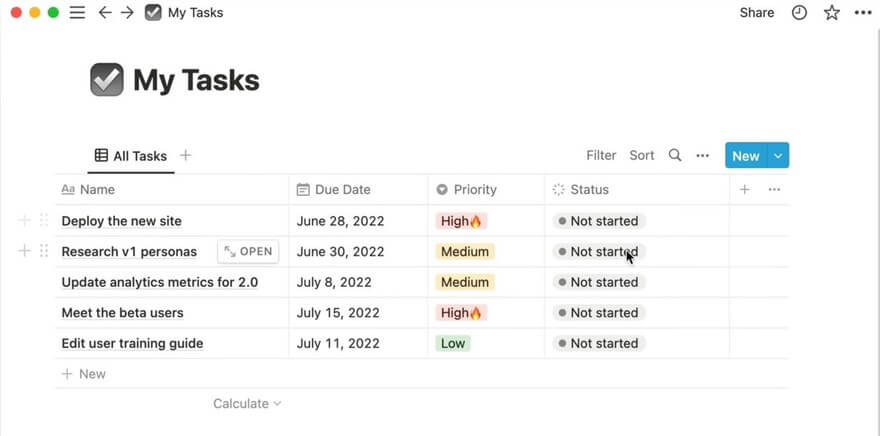This is a screenshot taken from a computer screen displaying a task management interface. The interface features a clean, white background with a gradient black-to-grey square that has a white gradient checkmark. The screen displays a task list titled "My Task," organized into five columns: Task Name, Due Date, Priority, Status, and Additional Actions.

Each column categorizes the tasks as follows:
1. **Task Name**: Lists the specific tasks to be completed.
2. **Due Date**: Shows the deadlines for each task (e.g., June 28th, June 30th, July 8th, July 11th, July 15th).
3. **Priority**: Indicates the importance of each task with options such as High, Medium, and Low.
4. **Status**: Displays the current status, with all tasks marked as "Not Started."
5. **Additional Actions**: Options to share tasks, set alarms, and star tasks for later prioritization.

The tasks listed include "Deploy the new site," "Research," "Update analytics," "Meet beta," and "Edit training guide." Users can sort and build this task list as needed, providing a comprehensive view for better task management and prioritization.